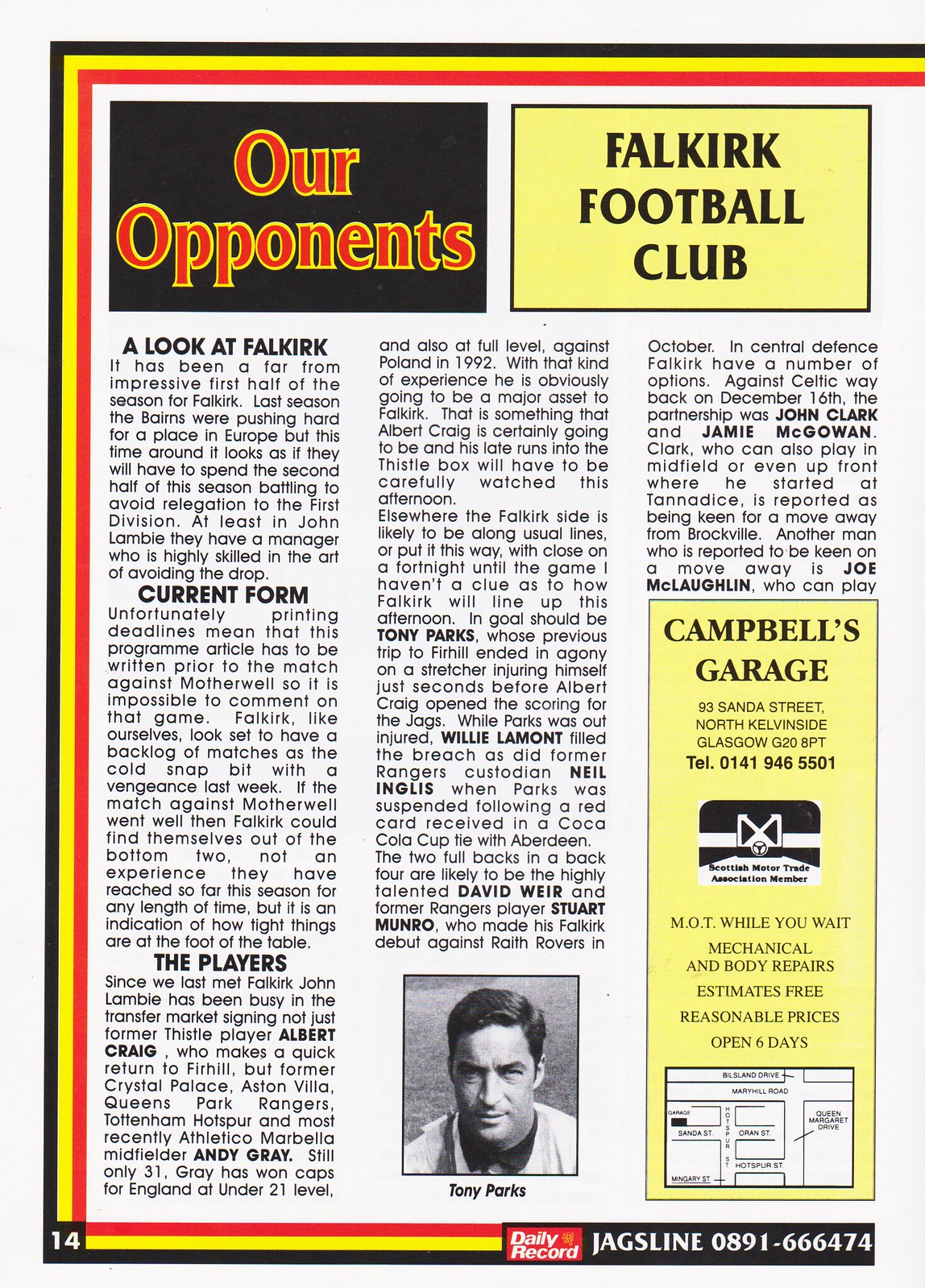This page from a British football club magazine, titled "Our Opponents," features a detailed analysis of their next adversary, the Falkirk Football Club. Positioned in the top left, a black text box with red text introduces the section, while to its right, a yellow text box with black lettering highlights Falkirk Football Club. The page is framed with three borders in black, yellow, and red. The main content is organized into three columns: the first section begins with 'A look at Falkirk,' followed by 'Current Form,' and 'The Players.' In the middle column, at the bottom, there's a black and white photograph of a player identified as Tony Parks. Adjacent to this, the third column features an advertisement in a long, yellow text box for Campbell's Garage, a mechanical and body repair shop. The page is marked as page 14 at the lower left corner, and includes a notation indicating it is part of 'The Daily Record Jags Line.'